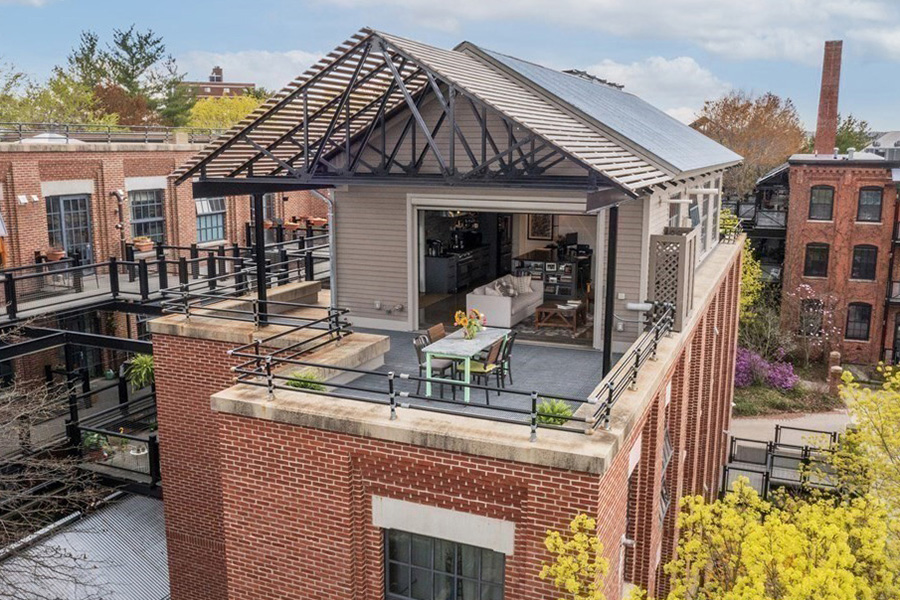This image depicts a vibrant, sunny neighborhood featuring charming, converted factory- or loft-style, two-story brick buildings adorned with modern additions. The central focus is a brick apartment with a white-roofed terrace, equipped with solar panels and encircled by black metal railings to ensure safety. The terrace boasts a light green table and chairs, along with a vase of flowers, creating a cozy outdoor dining area. Through an open garage-style door, a white couch and media storage unit are visible inside the apartment, suggesting a blend of indoor and outdoor living spaces. Surrounding this building are similar brick structures, complete with long windows and additional terraces. To the back left, a three-window brick building and lush trees are seen, while to the right, another structure with six windows and a prominent smokestack stands out. The ground level features gardens brimming with yellow forsythias, greenery, and various plant life, contributing to the neighborhood's vibrant and welcoming atmosphere. Bright blue skies with a few clouds complete this picturesque scene.